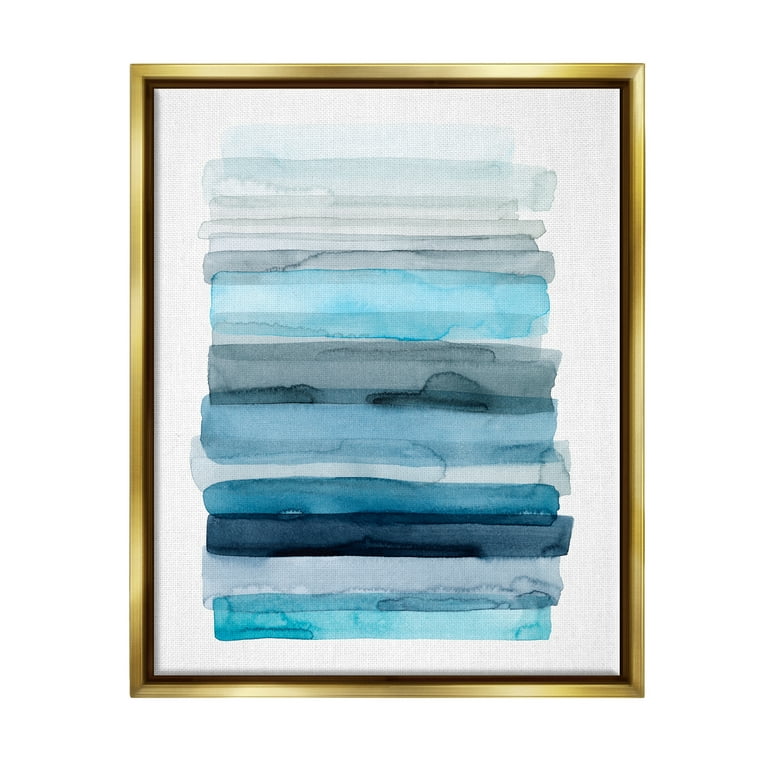The image is an abstract watercolor painting, framed in a golden frame with a thin brown inner border. The painting features horizontal bars in a range of blue shades, transitioning from light to dark, with some aquas and grays interspersed. At the top, there are lighter blue and grayish bars that gradually shift into medium blues, dark aquas, and nearly black hues towards the bottom. The bars eventually return to lighter blue and turquoise tones. The background of the painting is white, creating a striking contrast with the horizontal bars that appear to be randomly dripped and layered across the paper. The overall effect is one of stacked, semi-transparent layers, invoking a sense of fluid movement typical of abstract expressionism.